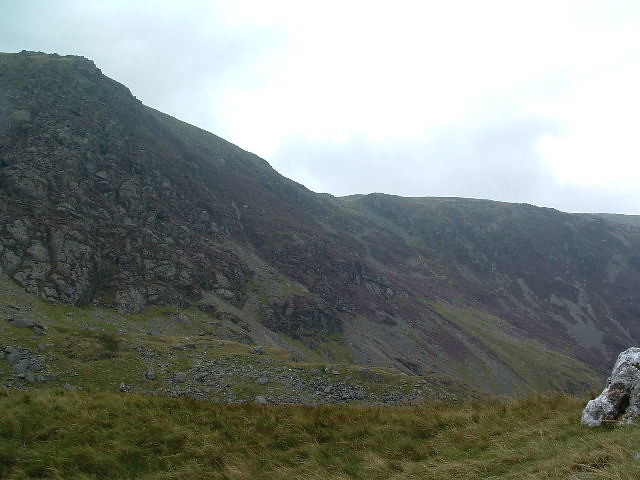The image depicts a serene mountainous landscape, captured from a grassy meadow. In the foreground, the bottom third of the image is dominated by lush, unkempt green grass, interspersed with gray rocks, including a notable small gray rock positioned in the lower right corner. Transitioning to the middle third, rocky and craggy mountain peaks loom, characterized by a mix of dark grayish-brown and black exposed surfaces. The tallest peak rises prominently in the top left of the image. Completing the scene, the top third features a partly cloudy blue sky, with patches of white clouds floating gently, suggesting a bright, sunny day. The overall composition indicates a remote, natural setting, possibly within a rugged mountain range.